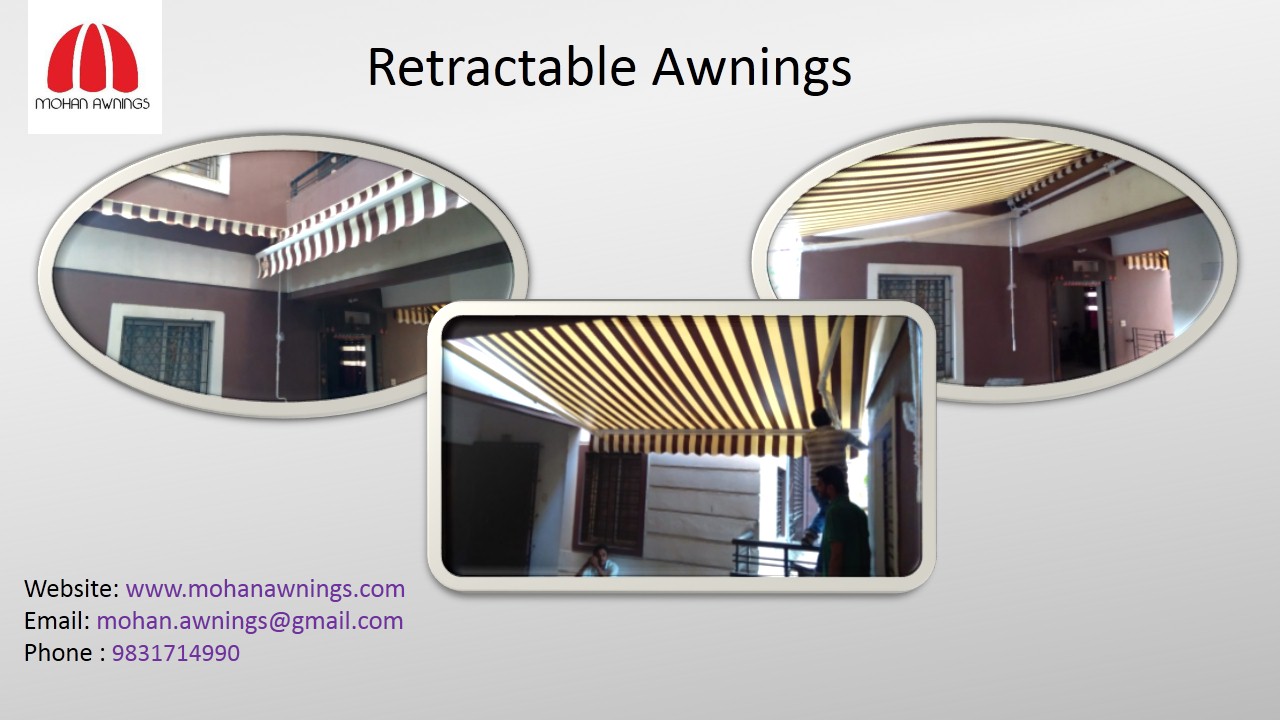The image is a detailed advertisement for McCann Awnings, featuring three montages that showcase retractable awnings. The top portion of the ad displays "Retractable Awnings" in bold black lettering along with a clip-art drawing resembling an umbrella, under which the text "McCann Awnings" is written. The background of the ad is predominantly white.

There are three distinct photos: the central one is rectangular and depicts workers demonstrating the operation of the awning. The flanking photos are oval-shaped; these two show the awnings in use, extended over outdoor areas to provide shade. The awnings come in horizontal or vertical stripes of yellow and brown or black.

Additional information includes a website, an email address (noted to be a Gmail account), and a jumbled phone number, all located at the bottom of the ad. This composition effectively combines elements of demonstrating product usage with relevant contact information for potential customers.